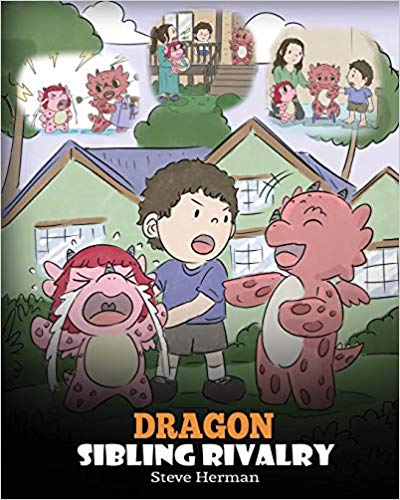The image resembles a children's book cover titled "Dragon Sibling Rivalry" by Steve Herman. It depicts a whimsical scene featuring two anthropomorphic dragons and a little boy. The dragon on the left, a pink creature with red polka dots, red hair, a white belly, and a pink tongue, is crying with white tears streaming down its face. In contrast, the dragon on the right, colored entirely in red with darker red polka dots and a white belly, is laughing. The boy, standing between them, wears a blue shirt, gray pants or shorts, white socks, and black shoes. 

Background details include a house with tanned walls, brown trim, and windows, topped with a black or gray roof. Green bushes span across the front, bordered by a grassy area, with trees featuring green leaves and brown trunks in the distance. The sky is a whitish-gray adorned with fluffy white clouds. Additional illustrations at the top left corner show the dragons against a white background, while the right corner features the mother, son, and dragons. Central to these images is a depiction of the house's porch, complete with brownish stairs and railings. The title "Dragon" is displayed in yellow, while "Sibling Rivalry" and the author's name, "Steve Herman," are written in white at the bottom.